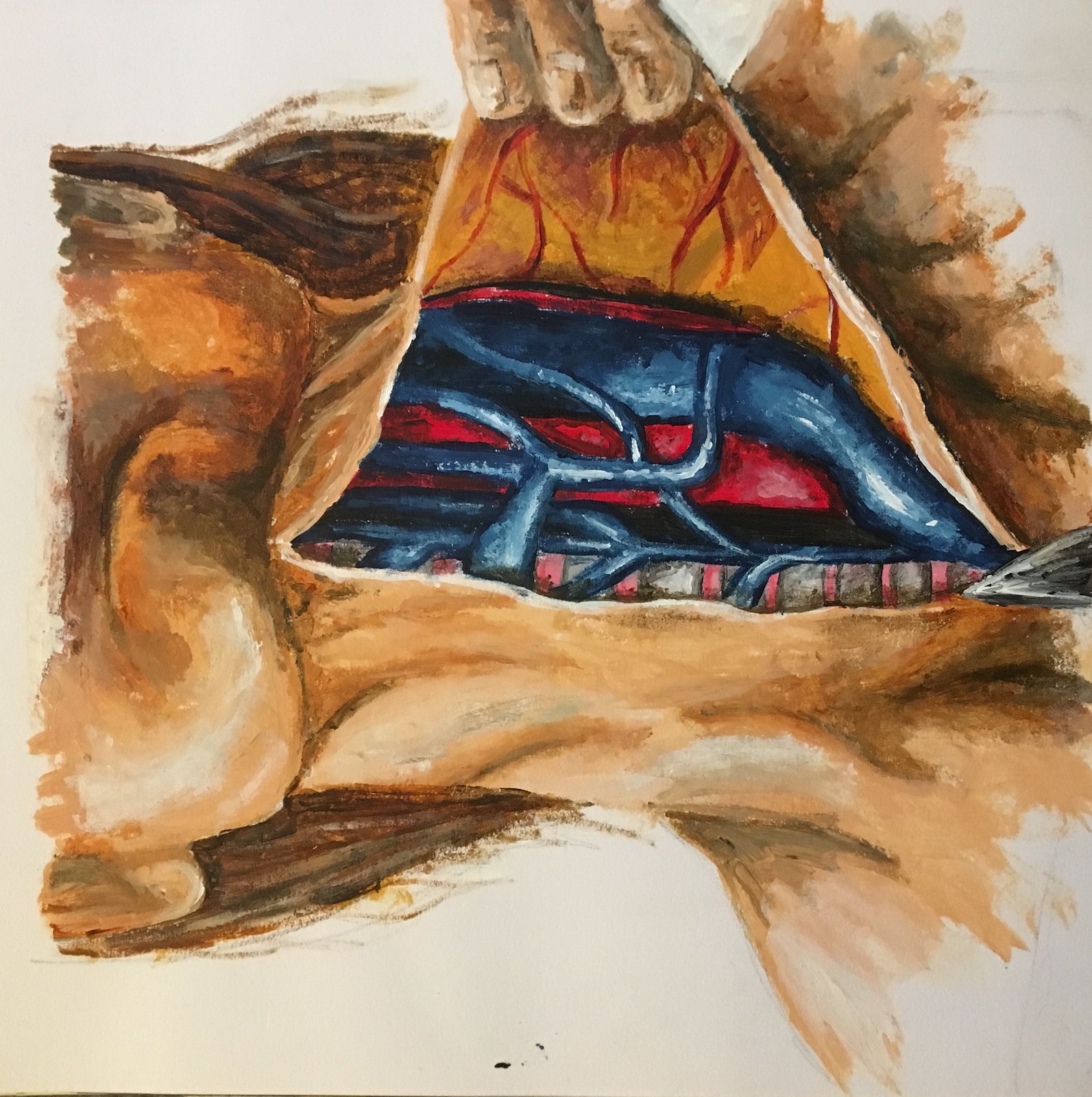In this detailed pastel artwork, the focus is directed towards the lower face, neck, and upper chest of a human subject, oriented horizontally with the head positioned to the left and the chest extending to the right. The depiction is meticulous, primarily in muted tones accented with blue and flesh hues. A set of fingers emerge from the top of the image, artfully pulling back the skin from the subject's neck. This reveals intricately detailed blue structures that resemble arteries, intricately winding beneath the surface, while glimpses of bone are visible, possibly representing portions of the spine. The juxtaposition of anatomical realism and artistic interpretation is striking. The subject's hair, which appears to be medium to long in length, cascades in fine strokes of brown. The complexion of the subject's skin is rendered in shades that suggest a white or tan ethnicity, adding to the lifelike quality of the piece. Overall, it's an evocative and visually arresting representation, blending elements of human anatomy with a surreal, almost clinical exploration of the body's inner workings.